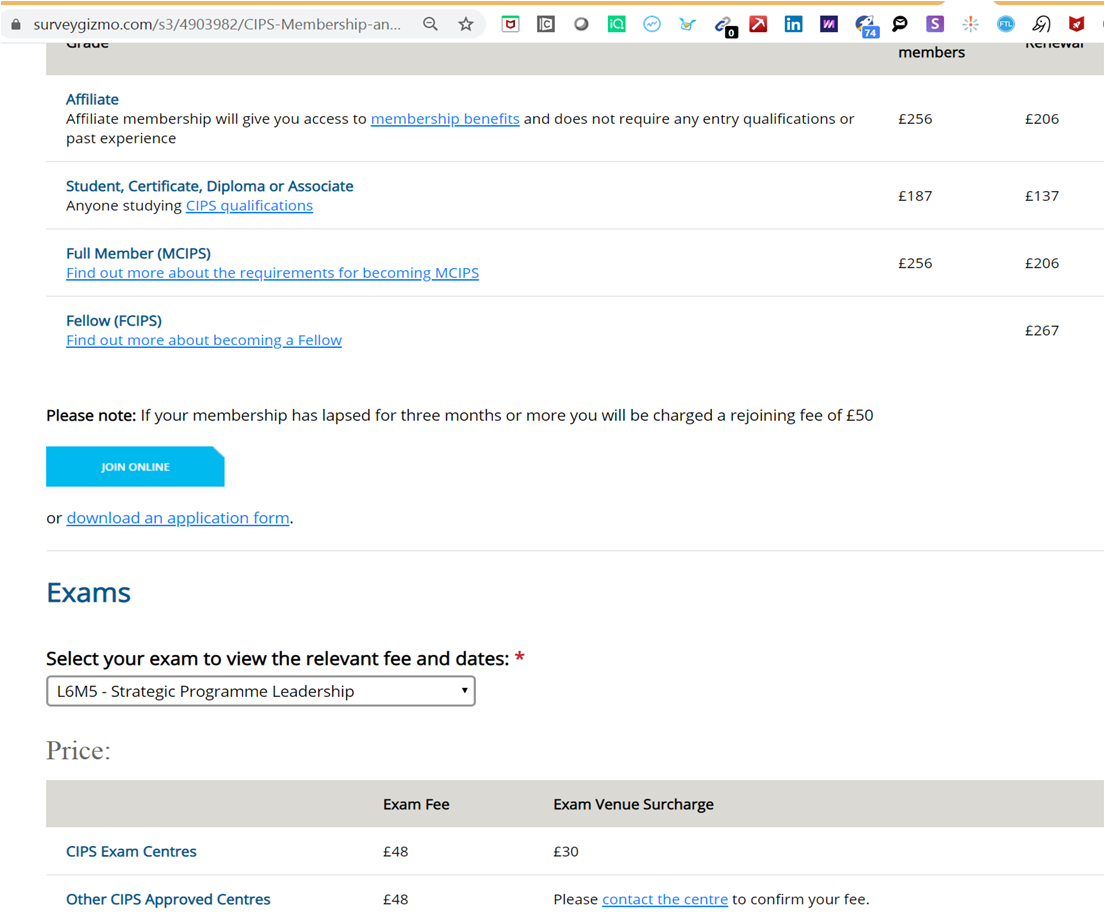This is a detailed screenshot of a webpage from SurveyGizmo.com, featuring an interface with a collection of various app icons at the top. The icons represent different applications, including McAfee and an app symbolized by a red box with a white pickaxe.

Below the icons, the page presents a membership selection interface with four categories: Affiliate, Student, Certificate/Diploma/Associate, Full Member, and Fellow. Each membership type comes with distinct benefits and pricing. The Affiliate membership, underlined by a highlight, offers access to member benefits without needing any specific entry qualifications or past experience. It is priced at £256 for new members and £206 for renewals.

Subsequent membership options are displayed with their corresponding prices, all under £300. The highest listed price among these options is approximately £267. A 'Join Online' button is prominently displayed for users to proceed with their membership selection.

Further down, there's an examination section that allows users to choose their exam and view the related fee schedule. This schedule includes two fees: an 'Exam Fee' and an 'Exam Venue Charge,' detailing the costs associated with taking the exam.